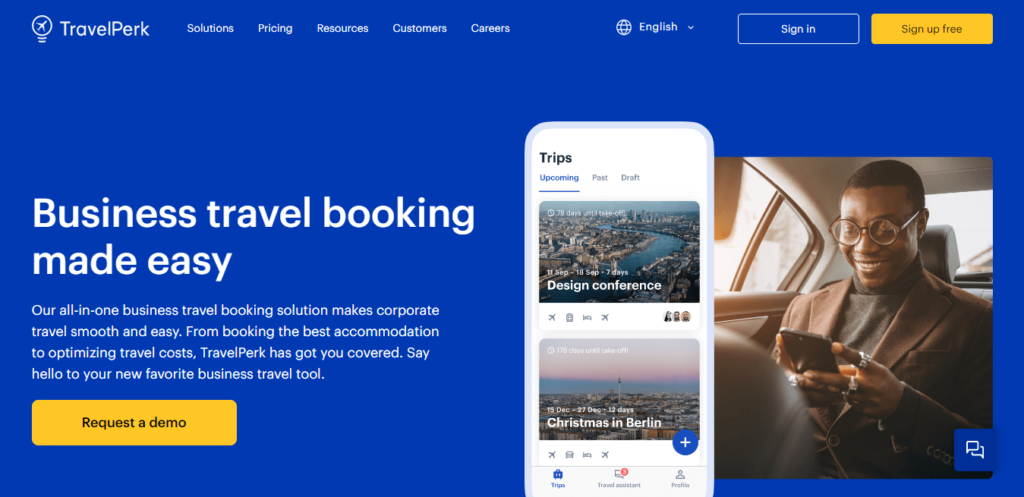The screenshot features the homepage of a website called TravelPerk, specialized in business travel solutions. In the upper-left corner, there's a logo depicting a small airplane encased within a circle, adjacent to the text "TravelPerk" in white font. To the right of the logo, a navigation menu offers various options: Solutions, Pricing, Resources, Customers, and Careers. Further to the right is a language selection tool, defaulting to English with other languages available. Next, there are two buttons for user access: a blue "Sign In" button with white text, and a gold "Sign Up Free" button with black text.

The overall background of the website is blue, with most text presented in white. In the center, a prominent gold button labeled "Request a Demo" with black text catches the eye, preceded by a headline in white reading "Business Travel Booking Made Easy." Below this, a brief white paragraph explains the service: "Our all-in-one business travel booking solution makes corporate travel smooth and easy. From booking the best accommodation to optimizing travel costs, TravelPerk has got you covered. Say hello to your new favorite business travel tool."

Embedded within this section is an image displaying a mobile phone showcasing two trip itineraries: "Design Conference" at the top and "Christmas in Berlin" below. Adjacent to this setup, there is an image of a man dressed in a suit, sitting in a car and smiling while looking at his phone.